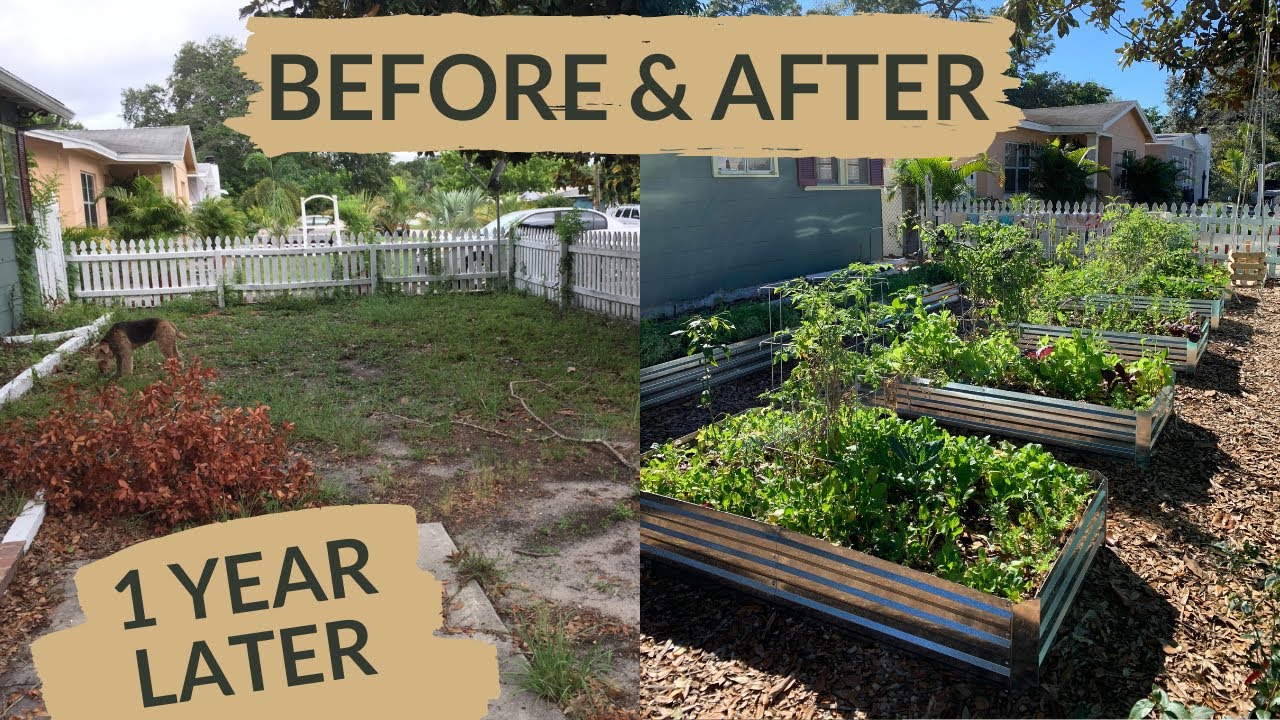This image, taken outside during the daytime, showcases a dramatic transformation of a backyard through a before and after collage. The yard is enclosed by a white picket fence and initially appears scruffy and barren, with a neglected patch of grass, a fallen tree branch, and scattered leaves, while a dog sniffs around the area. A small, withering bush stands amidst the untended lawn. The caption "one year later" appears at the bottom of the left photo, and above the entire collage, "before and after" is written in brown.

In the after image on the right, the backyard has undergone a significant makeover. Flower beds, constructed with sheet metal sides and wooden posts, are now teeming with lush greenery. The previously messy lawn is neatly covered with woodchips or mulch, enhancing the space's overall cleanliness and appeal. Additionally, small farming stations for herbs and spices have been set up, adding to the yard's charm and functionality. The transformation highlights the yard's shift from plain, brown grass to a vibrant, cultivated oasis.